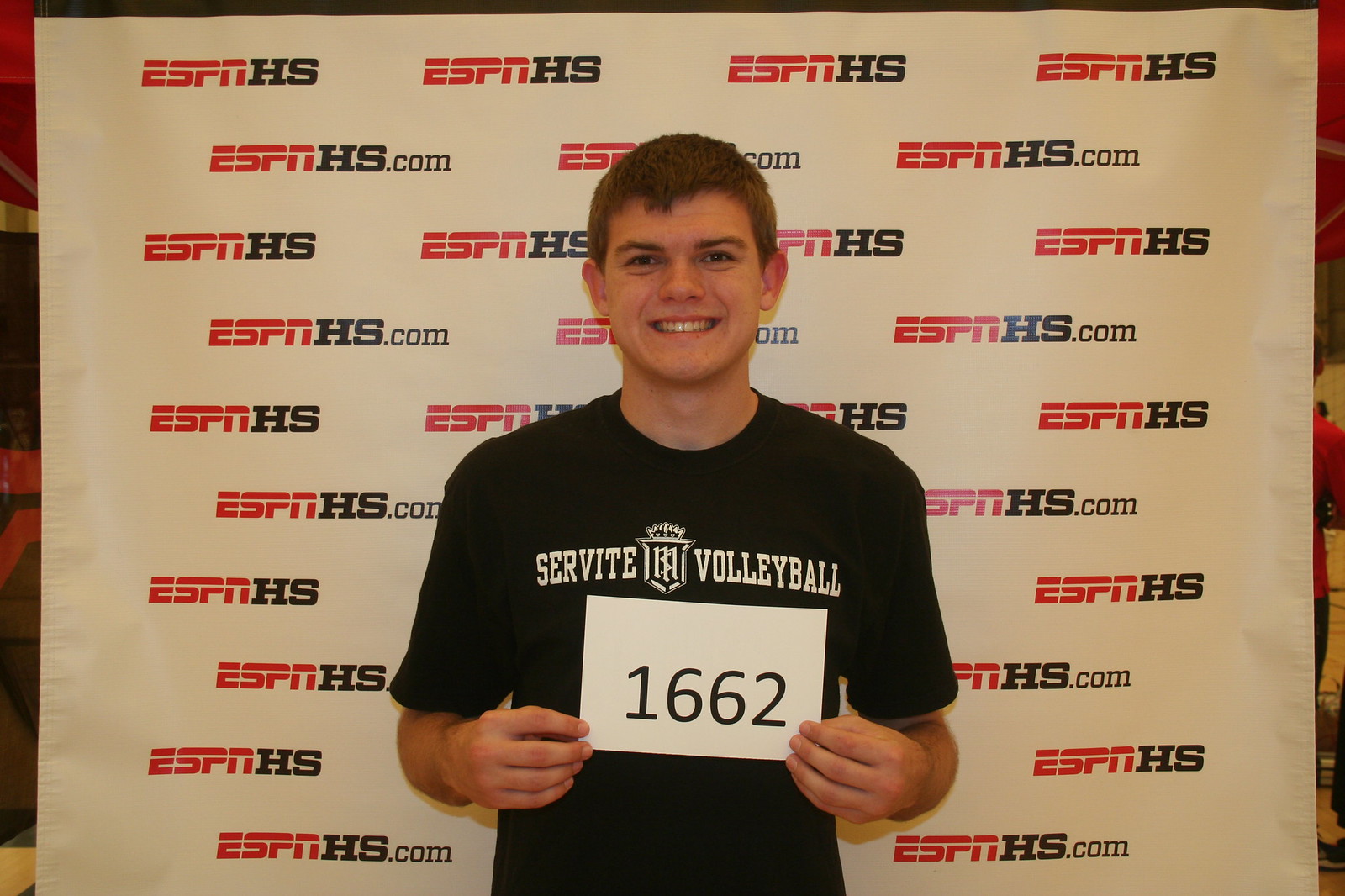The image features a smiling young man with short dark brown hair, standing in front of a white banner that repetitively displays the ESPN HS logo. The banner has rows alternating between "ESPN HS" and "ESPN HS.com" in red and black text. The man is dressed in a black t-shirt with white text that reads "Servite Volleyball" and a logo resembling a crown with an "M" inside it. He is holding a large piece of white paper with the black number "1662" printed on it, positioned just below the logo on his shirt. The overall context suggests a sports-related event, possibly involving volleyball, associated with ESPN HS.